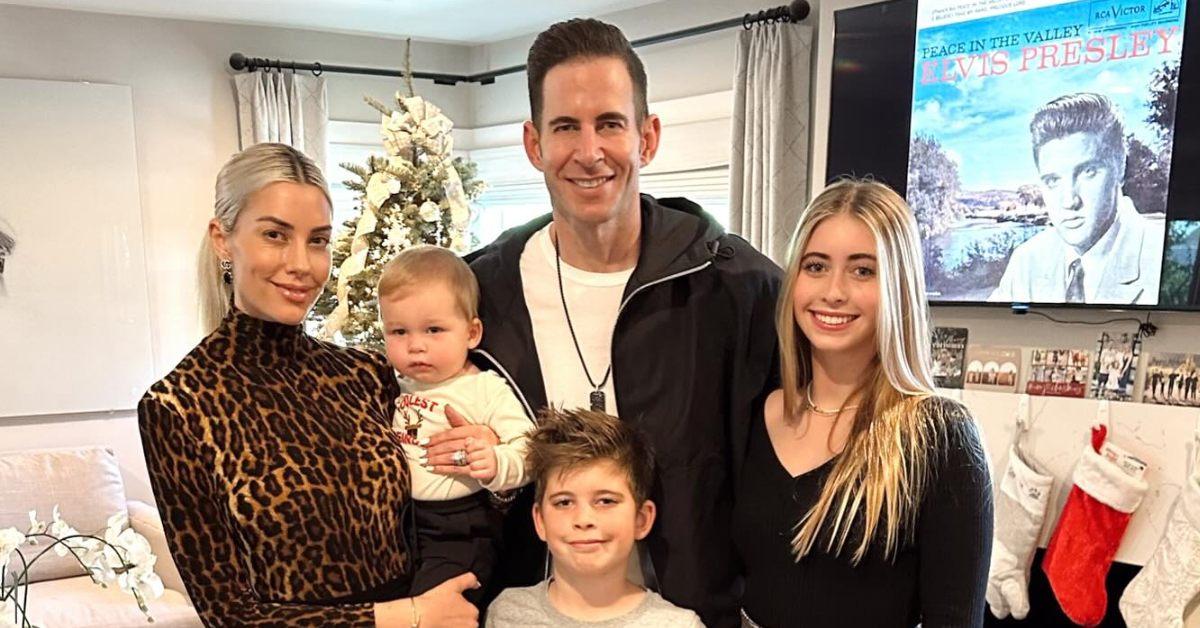This photograph captures a white family of five celebrating Christmas in their modern living room. Standing prominently is the father, Tarek, who is dressed in a dark gray zip-up windbreaker over a white t-shirt, with dog tags hanging from his neck. His new wife stands beside him, a blonde woman with her hair pulled back into a ponytail. She wears a long-sleeved leopard print top and earrings, and she holds their youngest child, a baby dressed in a white long-sleeved shirt and dark pants. To Tarek's left is his young daughter from a previous relationship, a blonde girl with her hair cascading down her back, clad in a black sweater and a necklace. In front of Tarek stands his son, a seven or eight-year-old boy sporting brown hair, a gray t-shirt, and a cheerful demeanor.

The setting captures the festive essence of Christmas, with a large green tree adorned with white ornaments like snowflakes and bulbs, and stockings—two white and one red—hanging from the mantelpiece. Behind them, a poster of Elvis Presley's "Peace in the Valley" subtly decorates the background, adding a touch of nostalgia. The warmth of family togetherness and holiday cheer is palpably depicted in this modern living room scene.